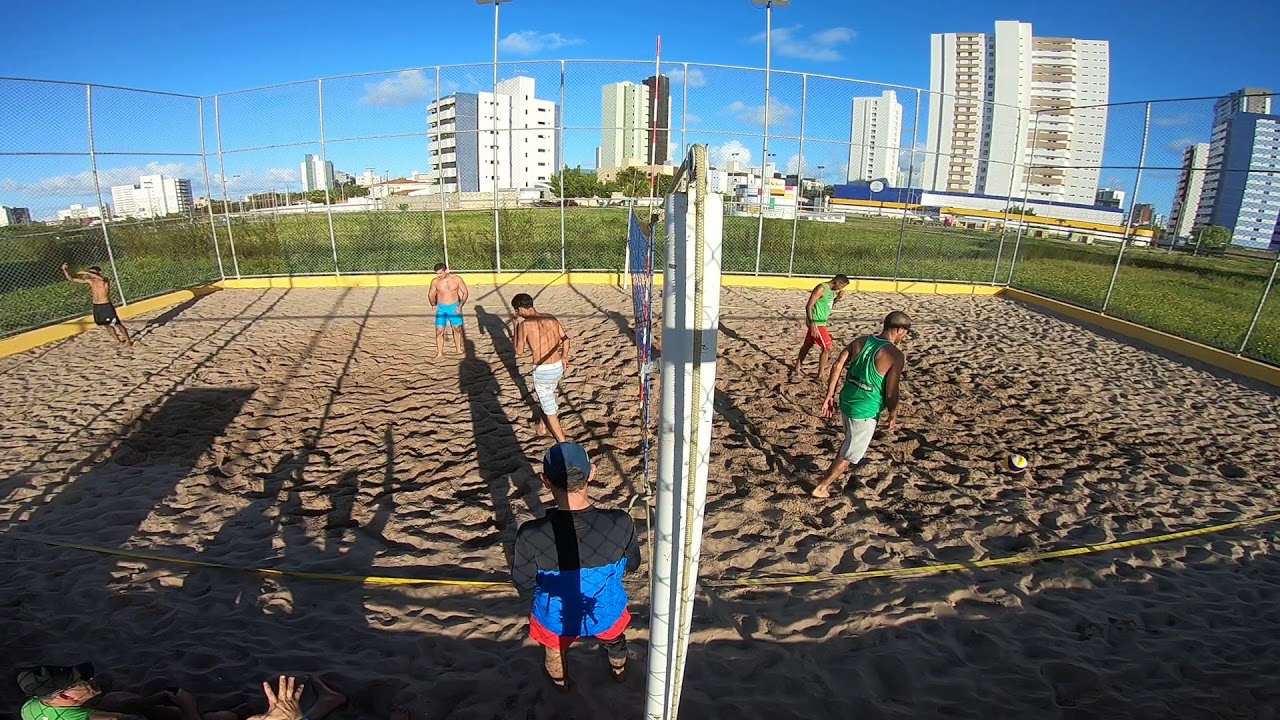The image depicts a lively volleyball game on a sandy court that is enclosed by a chain-link fence. The scene is bustling with activity, featuring six to seven men engaged in the game. The court is bordered by a yellow line, and a white volleyball net stands in the center. Among the players, two men wearing green tank tops are easily noticeable—one of them also wears red shorts. The players are a mix of shirted and shirtless individuals, with three men opting to go without shirts. In the background, a clear blue sky dotted with white and gray clouds stretches above. Surrounding the court, there is a lush green grass field and a variety of buildings. Tall high-rise complexes loom in the distance, interspersed with some smaller structures, lending an urban backdrop to this spirited outdoor scene.